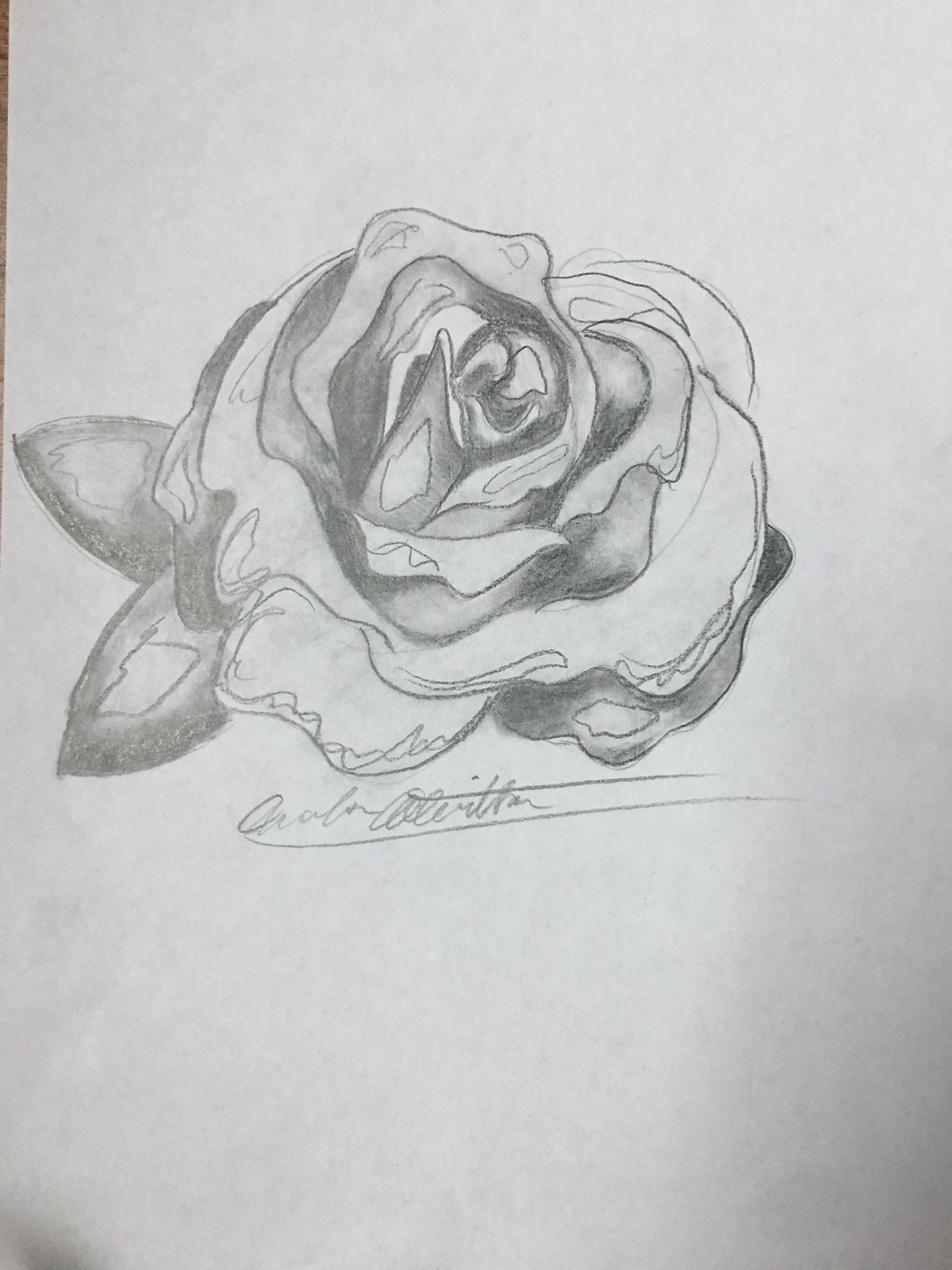This image showcases a detailed pencil sketch of a rose, created with what appears to be a standard number two pencil on an off-white sheet of paper. The drawing is vertical and spans a rectangular shape, capturing the intricate texture and delicate shading of the flower. The rose is centered on the paper and surrounded by two oval-shaped leaves with pointed tips on the left. The petals of the rose are meticulously detailed with numerous subtle lines and accents, indicating a high level of craftsmanship. The shading varies across the drawing, creating a realistic depth, with the inner petals shaded darker and outer petals lighter, giving a sense of dimensionality. At the bottom of the image, though partially obscured, is a cursive signature, underlined, presumably of the artist, starting with an indistinct letter, possibly 'A'. Shadowy areas, particularly at the bottom left and extending up from the bottom right, add to the naturalistic feel of the artwork, creating the illusion of depth and texture on the paper.